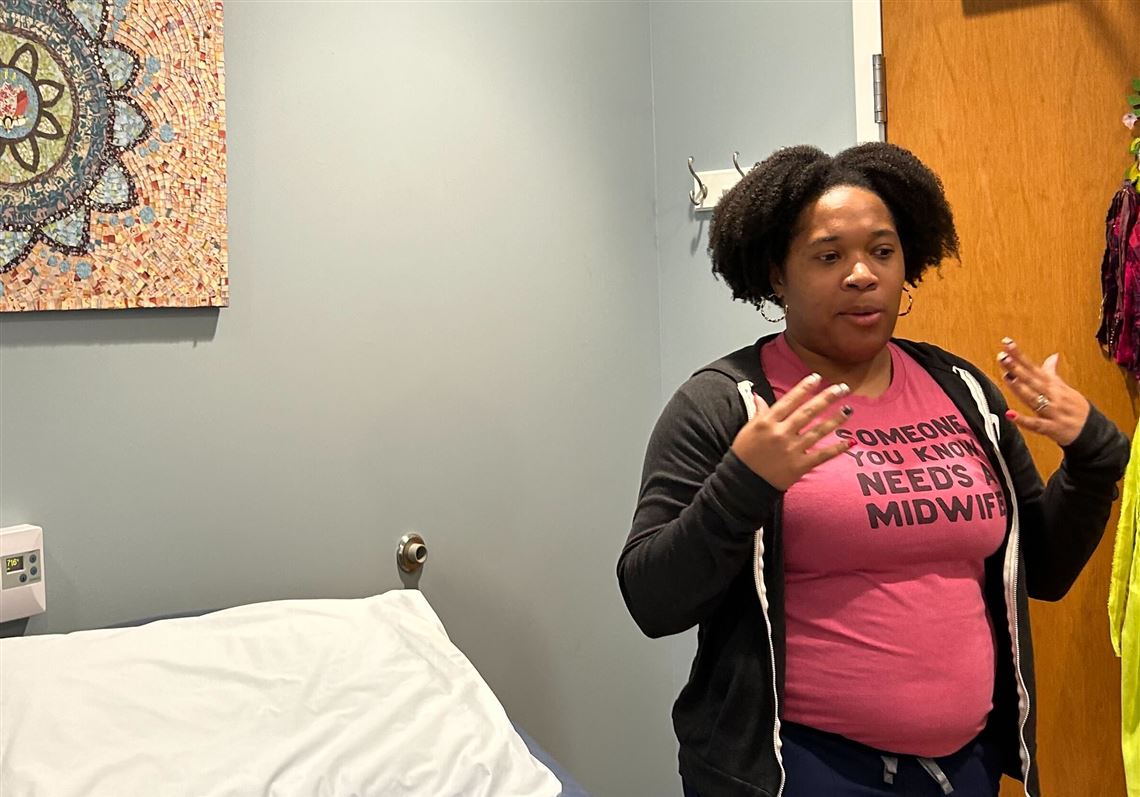The photograph features an African-American woman with dark skin and black curly hair, wearing a pink t-shirt that reads "Someone you know needs a midwife." Over her t-shirt, she has on a black hoodie with a white zipper. She is standing next to a bed, likely in a hospital or doctor's office, as indicated by the medical equipment, the bed, and the lighting typical of such settings. The walls of the room are light gray, and there is a brown door with a white frame visible in the background. On the wall to the left, there is a mosaic artwork depicting a flower. There is also a piece of wood with three hooks, possibly for hanging jackets, and a doorstop behind the door. The woman appears to be in mid-conversation or explaining something, with her hands raised, palms facing herself, suggesting an expressive gesture. She seems to be posing or possibly expressing surprise.